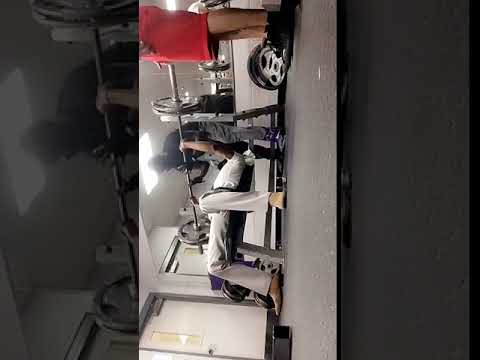In this color photograph, captured in portrait orientation and set within a larger, darkened landscape frame, a gym scene unfolds. A man, clad in a white t-shirt and gray pants with tan shoes, lies on a bench press machine, actively lifting a barbell. Above him, a spotter wearing a black sweater and jeans provides crucial support. To the right, another individual stands by, partially visible, dressed in red baggy shorts and black tennis shoes. The gym's gray flooring and overhead lighting are evident, with a large rectangular mirror behind the men, reflecting the active scene. Additional weights and gym equipment scatter the background, alongside a prominent white door.